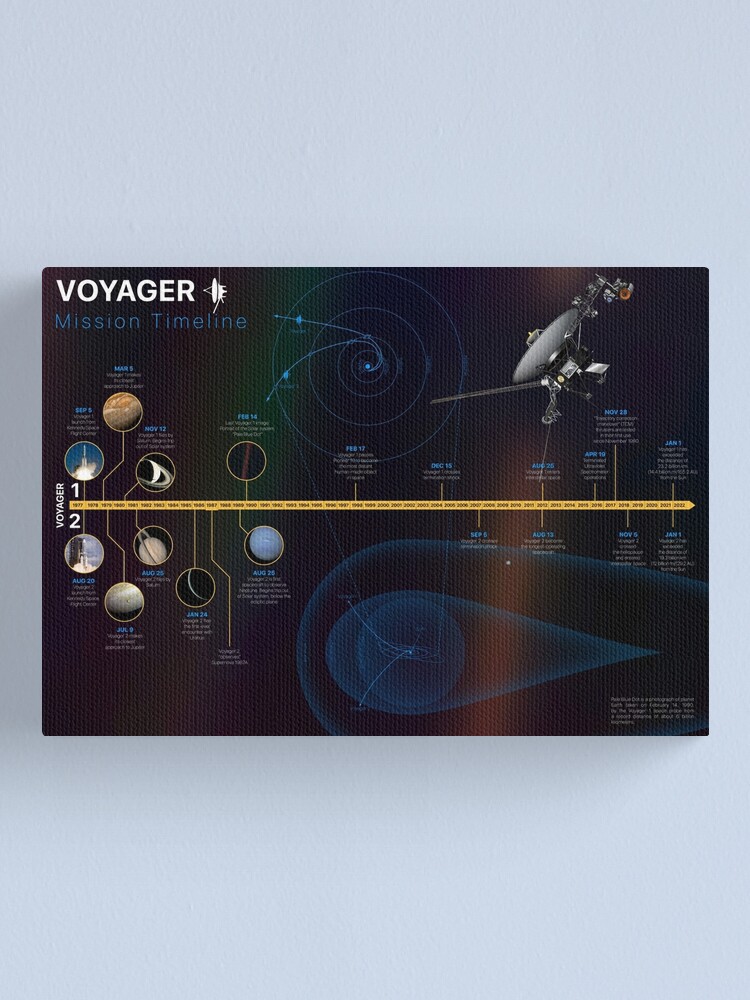This image is a detailed space-themed illustration titled "Voyager Mission Timeline," prominently displayed in bold white capital letters on the top left corner. It showcases a comprehensive timeline of the Voyager missions, marked from 1977 to 2022 in a thin yellow strip. The timeline features significant milestones, indicating key achievements and planetary encounters of the Voyager 1 and 2 spacecraft.

The illustration uses a color scheme of green, red, and yellow, with various circular icons representing different stages and encounters. A notable feature is a large circular light at the top, signifying a crucial event or milestone in the mission. Additionally, a satellite structure or spacecraft is depicted on both the top left and top right corners, one resembling a satellite dish that is typically used for television but is actually signifying the spacecraft and its journey through space.

The diagram includes a central bar running horizontally, illustrating sequential stages of the mission. Above and below this bar are small circles depicting planets and other celestial bodies like Mars and Saturn, indicated by specific visual cues such as Saturn's rings. Minimal text accompanies these circles, marking encounters and critical points of the Voyager missions. Overall, this poster effectively captures the significant events and the trajectory of the Voyager spacecraft in a visually engaging manner.